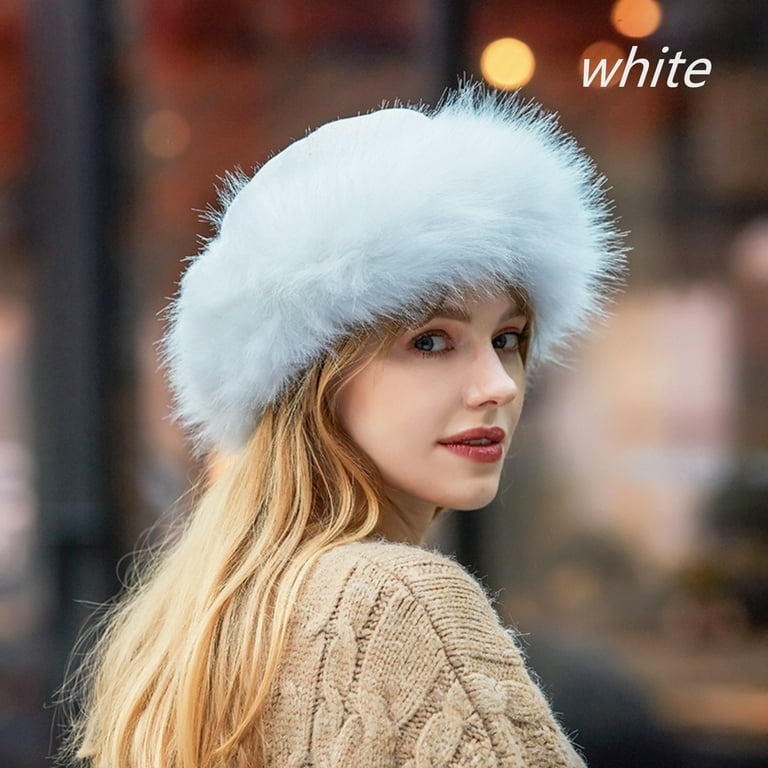In a professional portrait taken outdoors, a young Caucasian woman, likely in her 20s, stands against a blurred city street backdrop illuminated with urban lights. The image captures her from the shoulders up, highlighting her long blonde hair cascading past her shoulders. She wears a taupe, knitted sweater paired with a white winter hat featuring a fur edging, reminiscent of Russian styles. Her classic and light makeup includes mascara, light foundation, and striking red lipstick that complements her blue eyes. She glances over her shoulder towards the camera, her teeth just showing in a subtle expression. In the upper right-hand corner of the image, the word "white" appears in white italics, possibly indicating an advertisement for the hat.